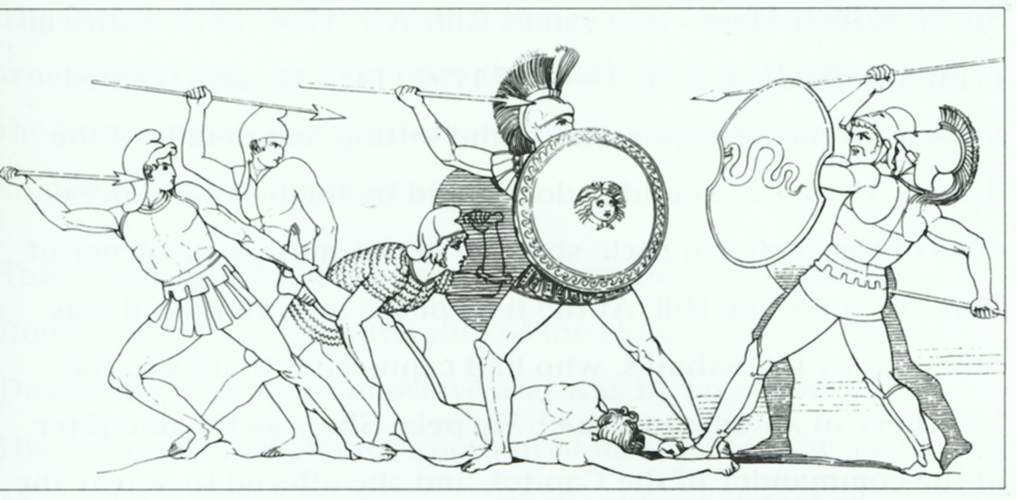This is a detailed black ink drawing, in a black-and-white color scheme, depicting an intense medieval battle scene. The scene features seven figures engaged in combat, with significant attention to detail and expressive line work. On the right side of the image, two fully armored warriors, each brandishing a spear in their right hand, are outfitted with shields adorned with a snake emblem. Opposing them are four men; three are standing upright with spears in hand, while one of these men is crouched, assisting in dragging an injured individual across the ground. This injured person is being pulled by the legs, likely to be moved out of the immediate danger. The shield on the leftmost warrior displays an intricate design of a woman or man with long hair, adding to the historical and artistic detailing of the piece. The emphasis on traditional combat gear and the vivid portrayal of each character's stance and equipment underscores the dynamic and chaotic nature of the depicted skirmish.